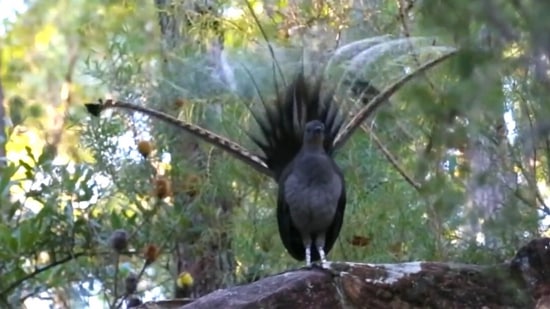The photograph is a full-color, rectangle image oriented horizontally. It captures a scene in a forest area during the daytime, featuring lush green foliage and various tree trunks in the background, which are slightly blurred, emphasizing the subject in the foreground. The centerpiece of the photograph is a large black bird with distinctive white legs and ankles. The bird is perched gracefully on a rock. Notably, the bird has an impressive display of tail feathers that fan out behind it in a V-shape, appearing almost translucent, much like those of a peacock. The bird's plumage presents a mix of black, brown, and gray hues. Despite the captivating scene, the photograph is somewhat low in resolution, lacking sharpness and clarity. Overall, it captures a serene moment of a majestic bird in its natural forest habitat on a seemingly beautiful, sunny day.